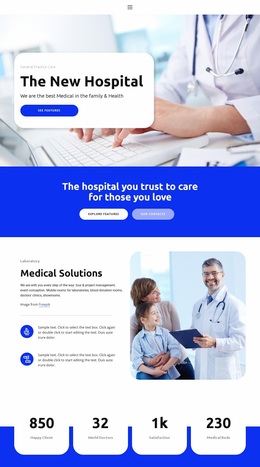This image is a composite screenshot divided into distinct sections filled with various details. 

At the top of the image is a square segment. The upper two-thirds of this square displays a photograph featuring a person's hands typing on a keyboard. The individual wears a white doctor's coat with a stethoscope draped around their neck, suggesting a medical professional at work.

Centered on the left within this square is a white rectangle with bold black text that reads "The New Hospital." Beneath this text is a line of smaller black writing, followed by a prominent blue rectangular button, though the button's text is not specified.

In the lower section of this square, set against a blue background, there is centered white text that says, "The hospital you trust to care for those you love." Beneath this text, there are two buttons centered on the screen: a white button on the left and a light blue button on the right.

Below this square, the background changes to white. On the left side, bold black text reads "Medical Solutions." Below this heading, there are three or four lines of smaller black text detailing more information, though the specifics are not provided. A thin white line separates this content from two blue icons stacked vertically. Each icon is accompanied by three lines of very small black print to its right, offering additional details.

On the right side of this white section is a photograph showing a male doctor, a woman, and a child seated on her lap, illustrating a caring medical scenario.

At the bottom of the image, there is a blue rectangle featuring four white squares, each missing its top side. Inside the first square, bold black text reads "850." The next squares show the numbers "32," "1k," and "230," respectively, likely indicating some statistics or metrics related to the hospital or healthcare services depicted.